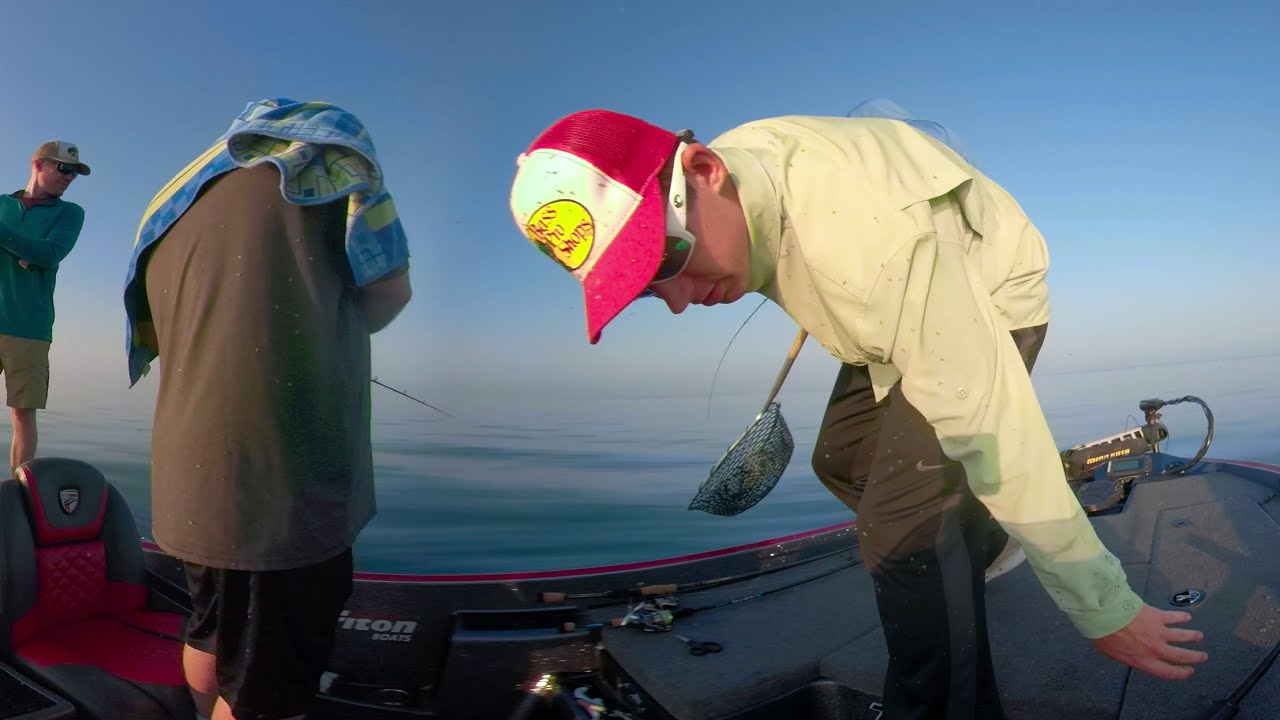A horizontally aligned rectangular picture captures a scene featuring three people on a red and black speedboat in the middle of the ocean. The background displays a clear blue sky with a few distant white clouds, and the gentle bluish-gray waves of water can be seen below. 

In the lower left corner, part of the boat's red and black seat is visible. Just in front of the seat, a man stands with his back to the camera, wearing black shorts, a brown t-shirt, and a yellow and blue towel draped over his shoulders, which obscures his head. To his right stands another man, identifiable by his red and white Bass Pro Shops ball cap, white sunglasses, and a long-sleeve light yellow shirt. He is leaning down to his left, stretching out his hand while holding a fishing net with a wooden pole in his other hand. He wears black and gray Nike athletic pants. A third man, positioned a bit further away on the far left, wears a brown and white ball cap with black sunglasses, a long-sleeve green shirt, and khaki shorts, appearing to look towards the water.

The calm atmosphere and soft lighting suggest it might be closer to sunrise or sunset, adding a serene quality to this dynamic fishing scene captured on open waters.